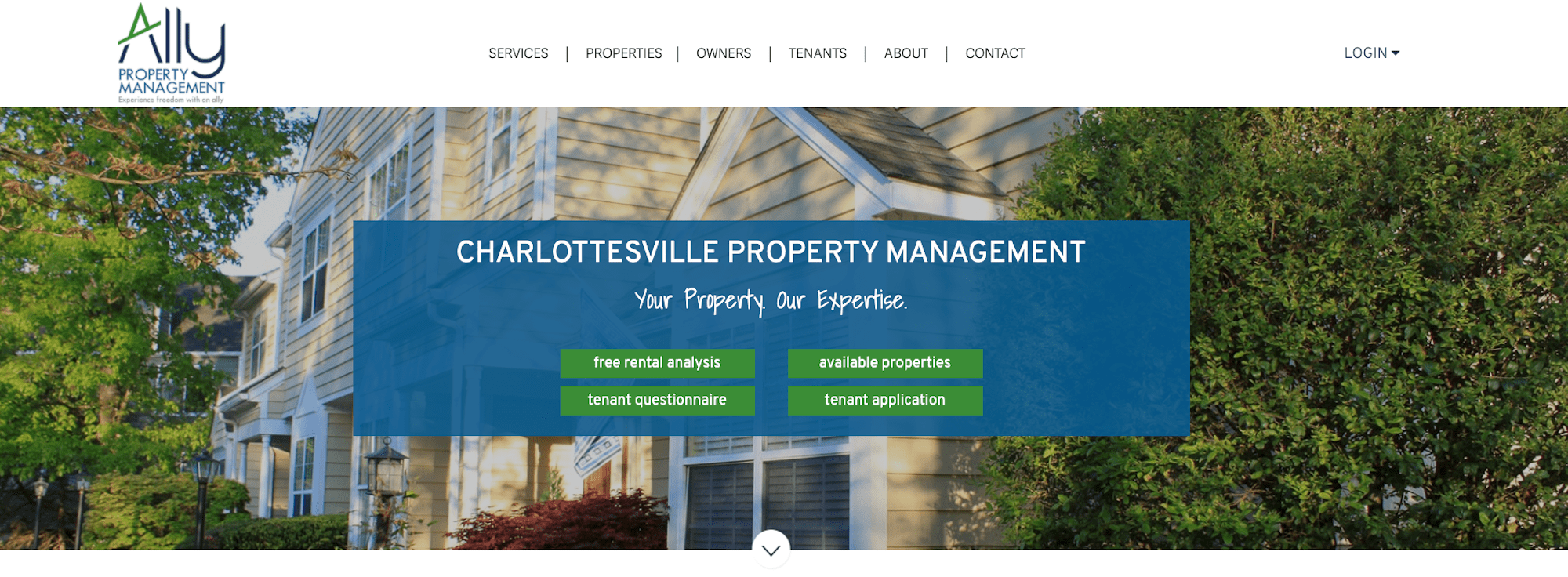The image depicts a beige house with white trim, flanked by trees on both sides, suggesting a serene suburban setting. The house appears to be constructed with vinyl siding. At the very top of the image, there is a banner that reads "Ally Property Management" with "Ally" in bold black letters and "Property Management" in blue lettering. 

Directly below this banner is a navigation menu with the following options: Services, Properties, Owners, Tenants, About, Contact, and Login, arranged horizontally across the screen.

Beneath the navigation menu, the main focal point is a beige house surrounded by greenery. Below the image of the house, there's a navy blue rectangle containing the text "Charlottesville Property Management." Below this, in smaller white letters, it reads "Your Property, Our Expertise."

Further down, the image features four green rectangular buttons arranged in two rows. The first row includes "Free Rental Analysis" and "Tenant Press Questionnaire." The second row contains "Available Properties" and "Tenant Application."